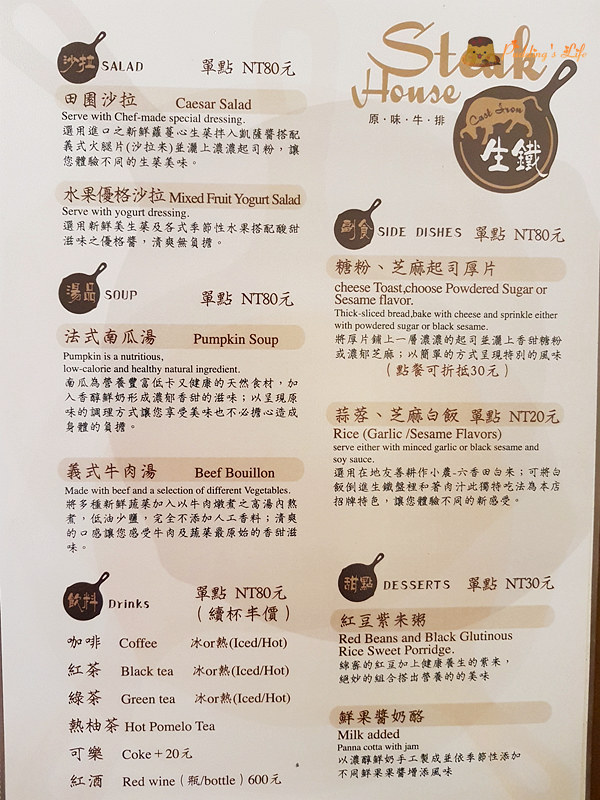The menu, for a steakhouse, is presented in both Japanese characters and English. At the top left corner, the section starts with "Salad," featuring options such as "Caesar Salad served with chef-made special dressing,” followed underneath by the same description in Japanese. The next item is "Mixed Fruit Yogurt Salad," also mirrored in Japanese.

An elegant design of an iron skillet serves as a divider. Below this, the "Soup" section offers a choice between "Pumpkin Soup" and "Beef Bouillon."

Following the soups, the "Drinks" section includes a variety of beverages: "Coffee," "Black Tea," "Green Tea," "Hot Pomelo Tea," "Coke," and "Red Wine."

On the right side of the menu, there is a "Side Dishes" section starting with "Cheese Toast," where you can choose between "Powdered Sugar" or "Sesame Flavor." The next side dish listed is simply "Rice."

Below the side dishes, the "Desserts" section features "Red Beans and Black Glutinous Rice Sweet Porridge" with a note that "Milk Added."

In the top right corner, the word "Steakhouse" is prominently displayed, accompanied by Japanese writing and symbols of a skillet, reinforcing the theme of the menu.